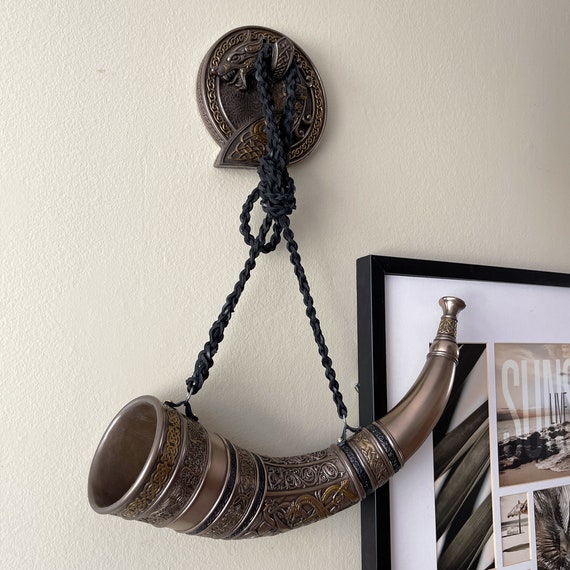The image features a detailed Viking-style drinking horn, prominently displayed on a cream-colored, textured wall. The horn has a rich brownish-bronze hue with decorative engravings and is shaped akin to an elephant tusk or battle horn. It is suspended horizontally by a black braided string from an ornate wall mount. The mount is a black, Dragon-themed medallion that resembles an Ouroboros, with the dragon's wings elegantly wrapped around its base, giving it a fantastical, Game of Thrones-esque appearance. Below the mounted horn, to the right, is a thin black-framed photo collage featuring beach scenes, further enhancing the decorative and homely ambiance of the setting.